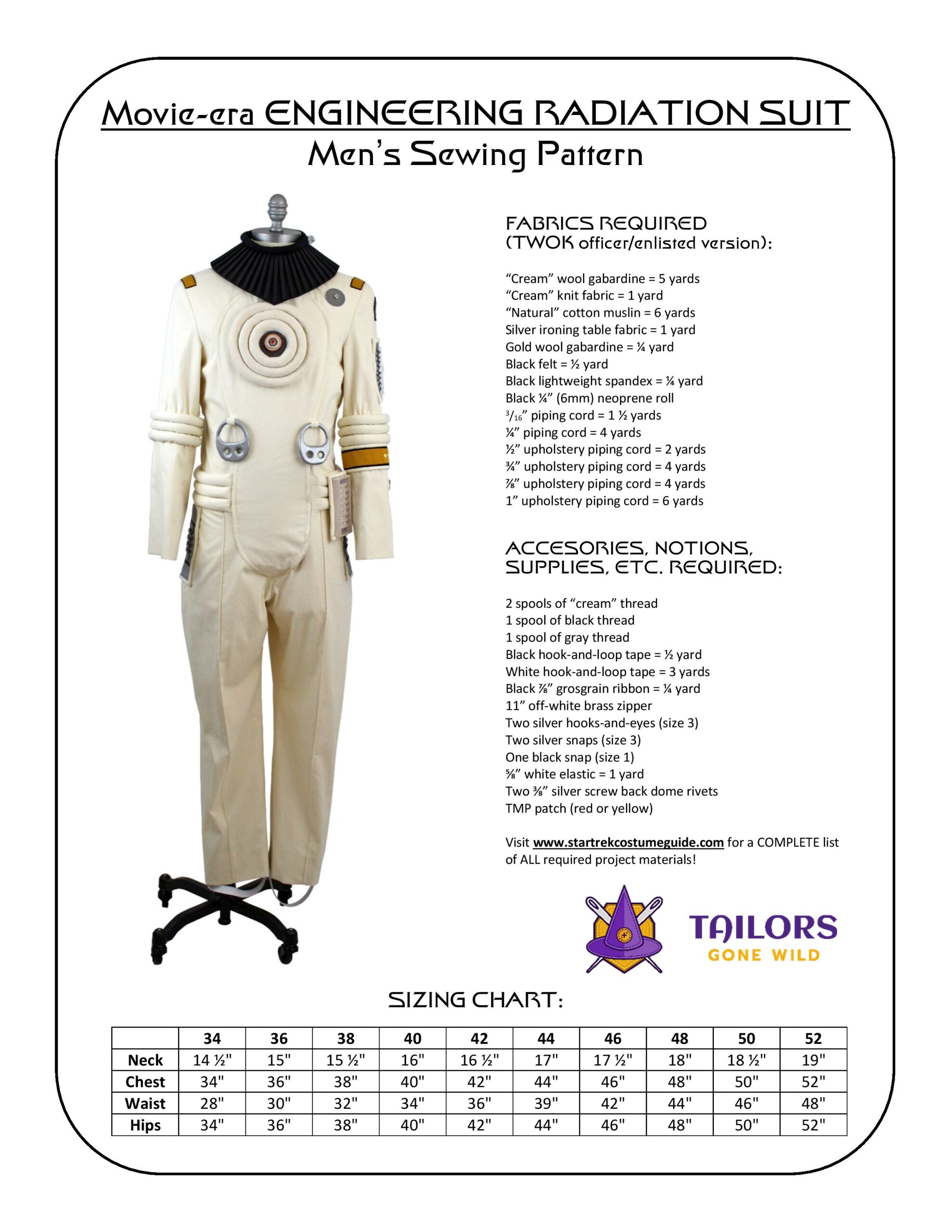This image is an instructional guide for sewing a "Movie Era Engineering Radiation Suit Men's Sewing Pattern." The guide is set on a white background with a rectangular shape and curved sides. At the top, in bold black text, the title "Movie Era Engineering Radiation Suit Men's Sewing Pattern" is prominently displayed. Below the title, on the left side, there is a visual of the actual radiation suit. This cream-colored one-piece suit features a black neckline, orange detailing, and silver accents. It has long sleeves with circular patterns on the sleeves and a gold strip and emblems on the left upper arm. The suit is displayed on a black stand with wheels.

On the right side of the image, there are detailed instructions, starting with a section titled "Fabrics Required," which lists specific materials needed for the "TWOK Officer Enlisted Version," including five yards of cream wool gabardine. Below this, another section titled "Accessories, Notions, Supplies, etc. Required" outlines additional materials necessary for the construction of the suit.

At the bottom of the image, a logo in purple and orange reads "Taylor's Gone Wild," accompanied by a wizard hat emblem. Beneath the logo, a detailed sizing chart provides measurements for neck, chest, waist, and hips, with sizes ranging from 34 to 52. Additionally, a website URL, "www.startrekcostumeguide.com," is listed for a comprehensive list of all required project materials.